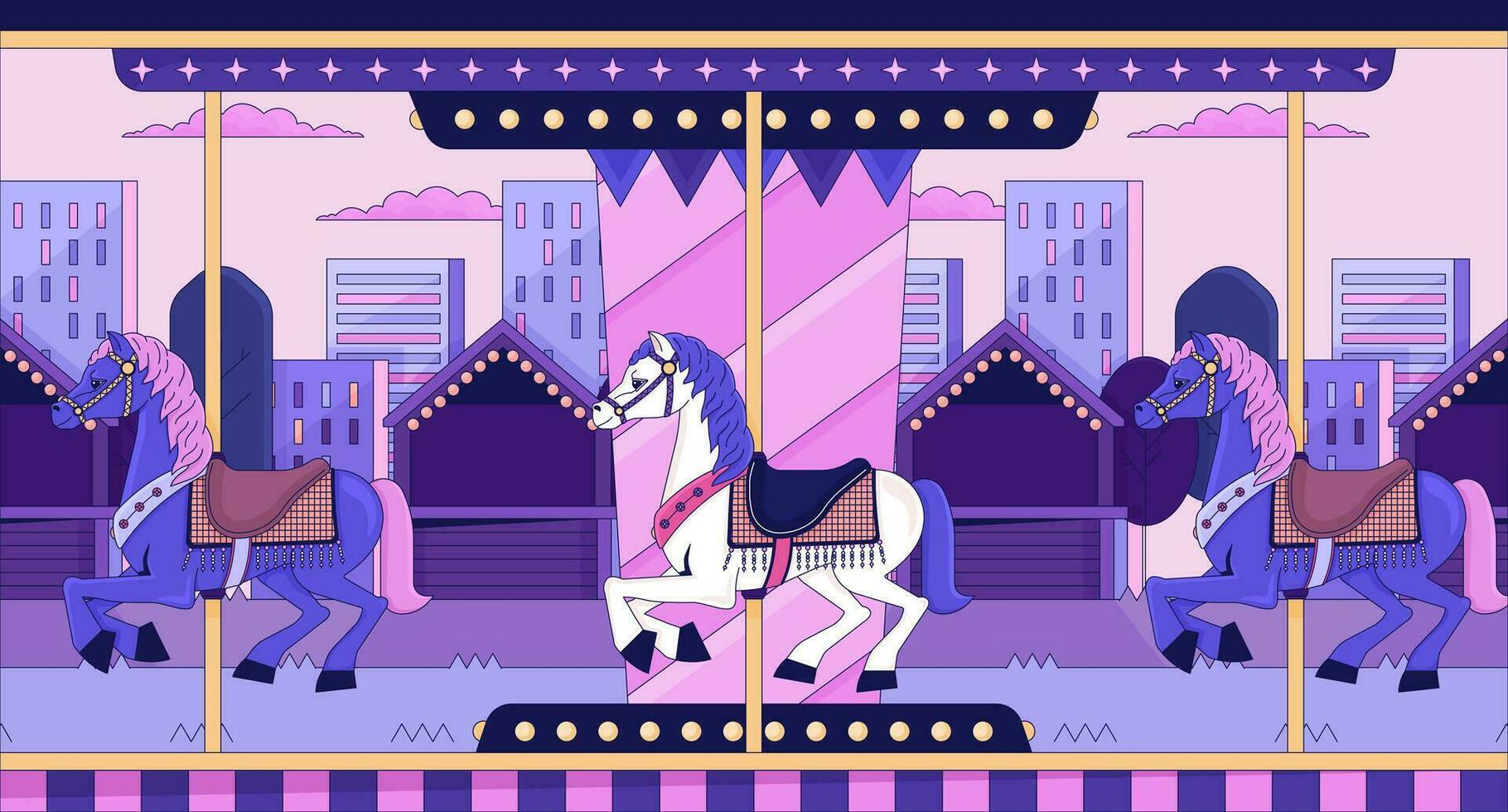This image showcases a vibrant, cartoon-style wallpaper border designed for a child’s room, depicted in a horizontal rectangle format. The border features a merry-go-round with three colorful hobby horses set against a whimsical cityscape. The predominant color scheme includes shades of purple, pink, and white, creating a fun and modern atmosphere.

At the top, the border is adorned with a black horizontal bar followed by a gold one. Below that is a purple strip decorated with white stars, then a narrower black bar studded with uniformly spaced gold dots. Blue and purple triangular pennants hang downward, alternating in color.

The main element features three hobby horses, each positioned on gold poles. The left and right horses are identical purple hobby horses with pink manes and tails, brown saddles, and gold bridles, depicted as if galloping. The central horse is white with a purple mane and tail, a black saddle with a brown saddle blanket, and a pink or dark pink martingale, also appearing in mid-gallop.

Behind the horses, there is a playful depiction of a carnival scene with purple string-lit kiosks that have dark purple shutters and purple brick bases. Above the kiosks, pink roofs with string lights form a festive atmosphere. Beyond this carnival setup, the background reveals a cartoonish city skyline with purple and pink skyscrapers and dark pink puffy clouds set against a pink sky.

The base of the border features another black bar with gold dots above a gold horizontal bar. Beneath the gold bar, a pink and purple striped banner completes the scene, adding a final touch of color and fun.